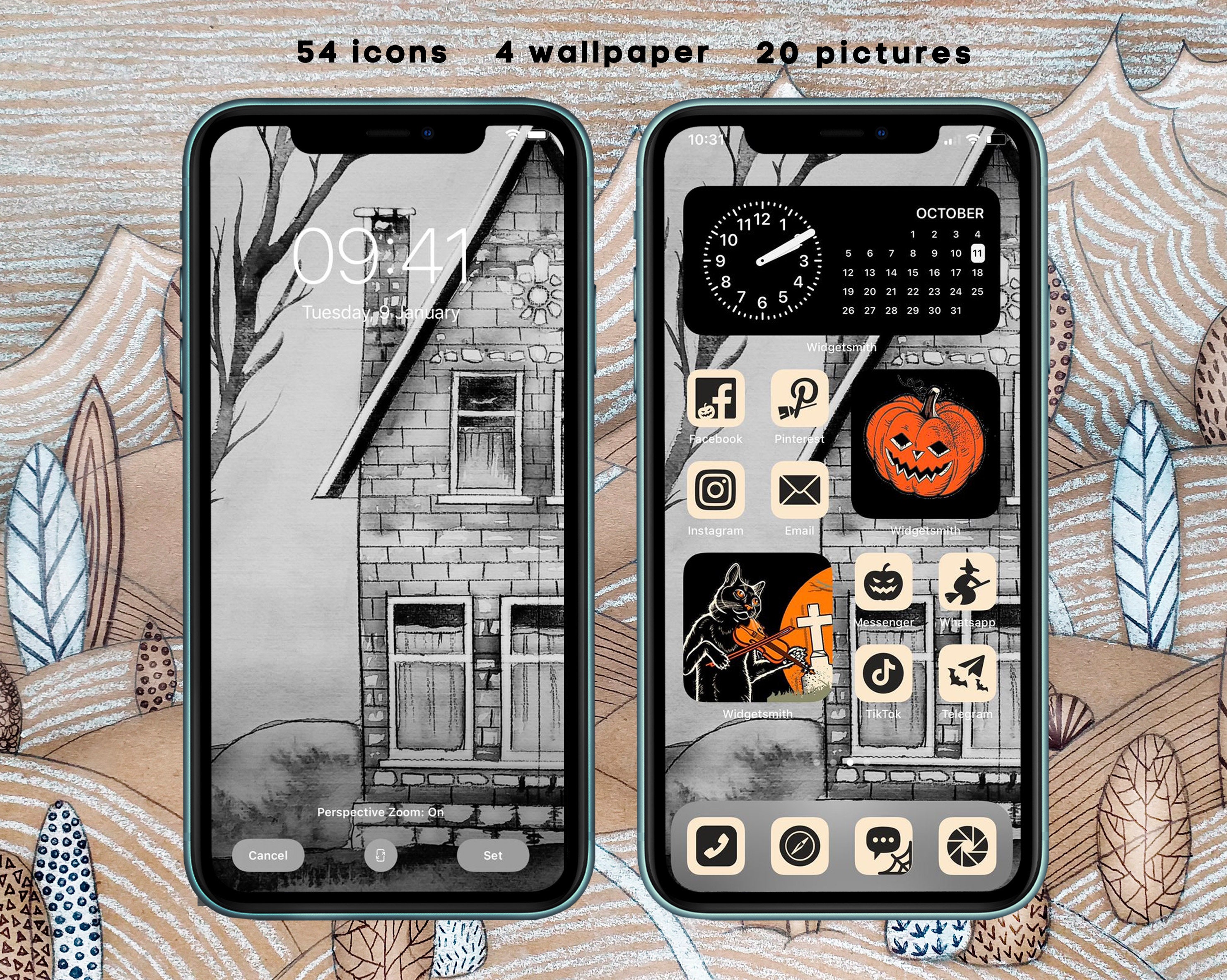The image is a screenshot featuring two smartphones placed side by side. At the top of the screenshot, there is text indicating "54 icons, 4 wallpaper, and 20 pictures." The phone on the left displays a lock screen with a digital clock showing the time as 9:41, and the date as Tuesday, January 9th. The lock screen features a black-and-white illustration of a cartoonish house.

The phone on the right reveals the home screen, which is adorned with multiple widgets and icons. At the top of this home screen, there is a widget that includes a clock on the left side and a calendar on the right. Below this, two additional widgets are visible: one displaying an image of a jack-o-lantern, and another featuring a picture of a cat.